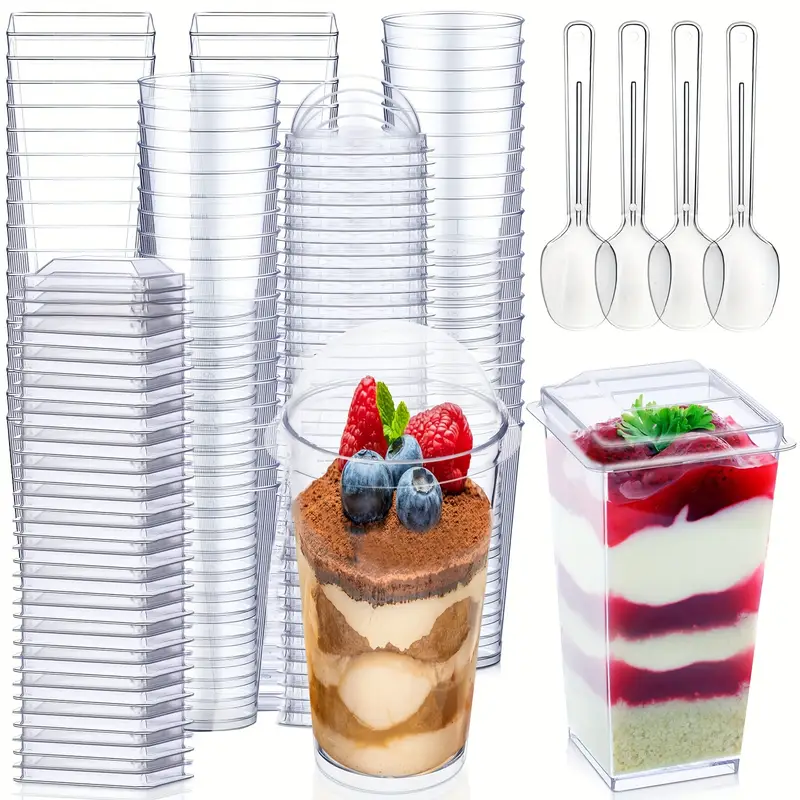The image appears to be an advertisement for plastic containers that includes a variety of clear, stackable plastic containers, both round and square, along with corresponding lids. The round containers feature domed covers, while the square ones have flat lids. The containers are arranged in vertical stacks, with separate stacks for each type of lid. In the upper right-hand corner of the image, four plastic spoons are hanging downwards, side by side. 

In the bottom center and bottom right of the image are two dessert parfaits - one in a round container and the other in a square one. The round parfait consists of layers of cream, brown crumbs, and fruit, topped with strawberries and blueberries. The square parfait features alternating layers of white cream and strawberry jam, garnished with green leaves. The image overall has a white background, making the colorful desserts and transparent containers stand out clearly.